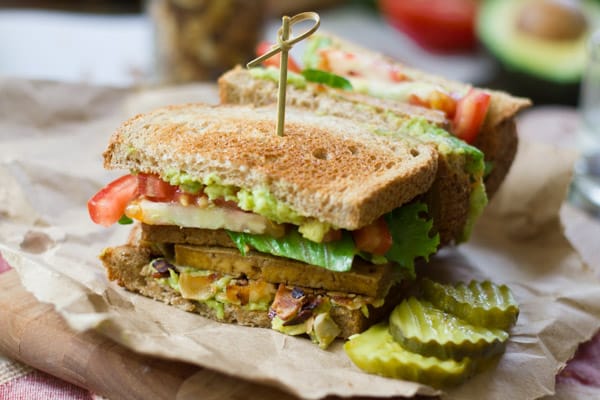The photograph features a detailed close-up of a club sandwich, meticulously presented on a piece of slightly torn, beige parchment paper, serving as a makeshift plate atop a brown wooden board. The sandwich, cut in half, is centrally positioned with one half standing on its side. The toasted bread is beautifully browned, securing layers of fresh ingredients. Visible fillings include crisp lettuce, juicy red tomato slices, creamy avocado mash, and cheese. Additional possible ingredients, suggested by some descriptions, include a brownish-yellow block presumed to be either tempeh, tofu, or maybe a layer of egg salad. A toothpick secured with a ribbon-tied bamboo sliver holds each sandwich half together. Nestled to the bottom right corner are three ridged pickle slices. In the softly blurred background, halved avocados with their pits intact and tomatoes add a touch of rustic charm to the overall composition.